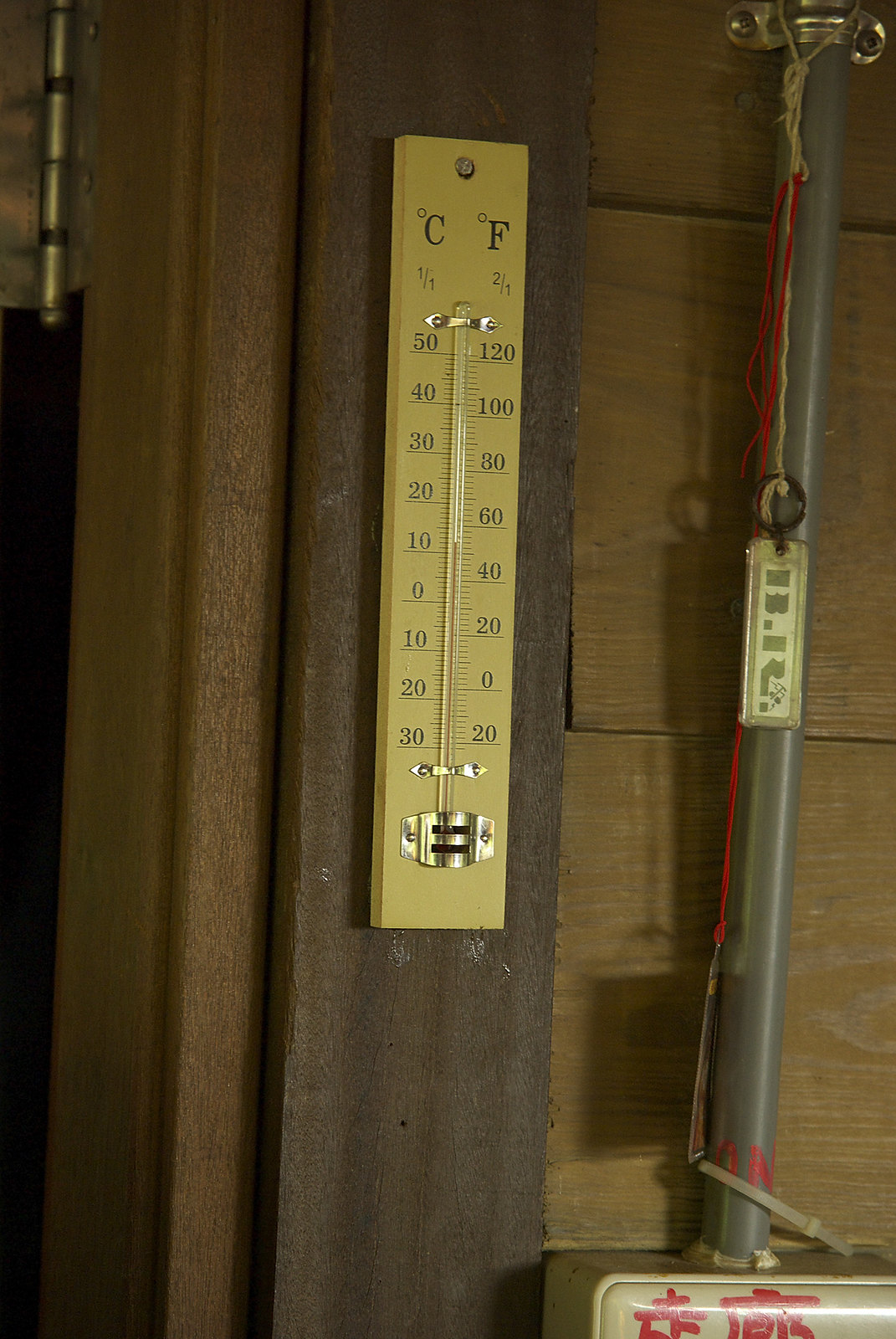This photograph showcases a yellow thermometer mounted on a wooden doorframe on the exterior of a house. The thermometer, which measures the outside temperature, displays readings in Celsius on the left and Fahrenheit on the right. The current temperature is slightly above 12 degrees Celsius (approximately 52 degrees Fahrenheit). The house’s siding, like the doorframe, is constructed from wood. Adjacent to the doorframe, a rod extends upward with several attached wires, primarily red, leading to the top. These wires originate from a partially visible metallic box on the side of the house, which features red Japanese lettering. Additionally, there is a tag affixed to the wires on the rod.